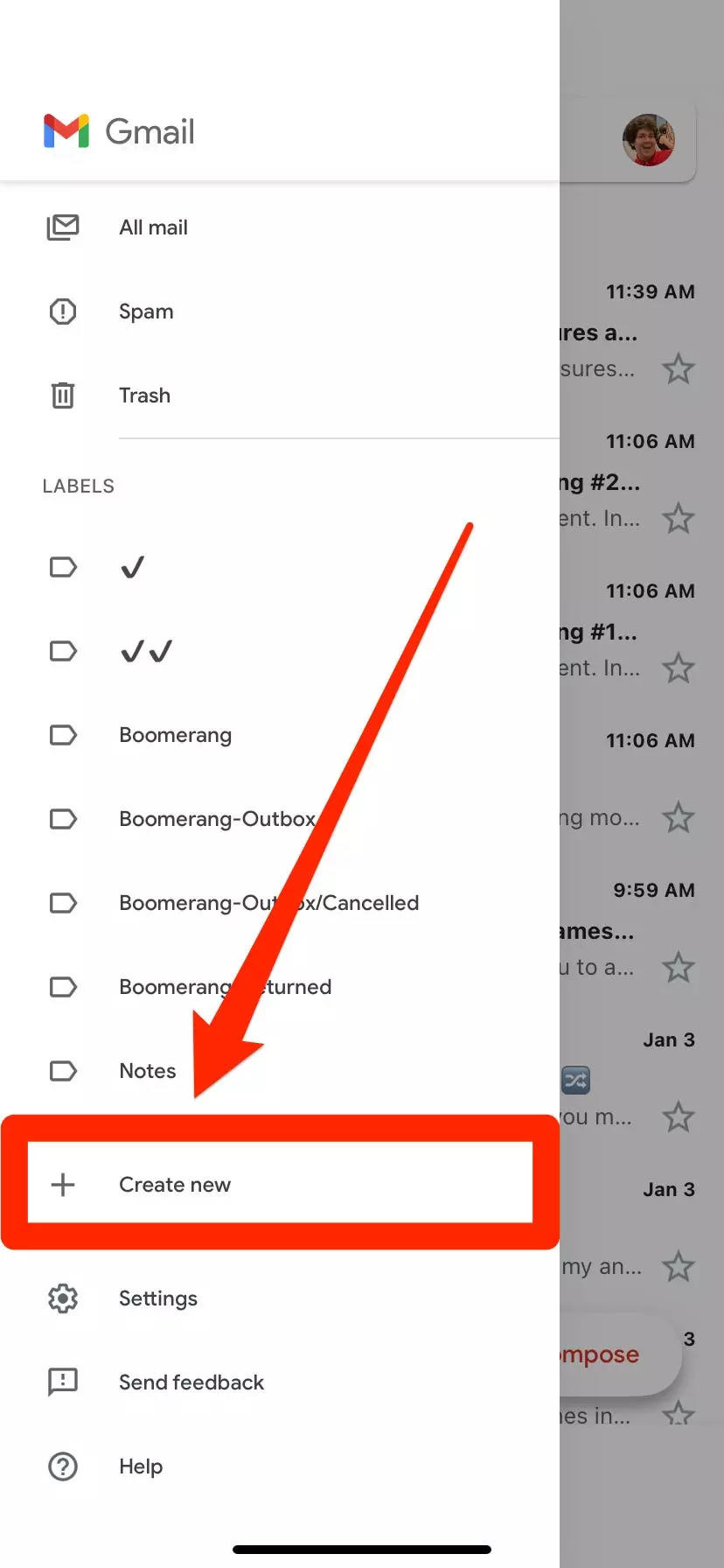The image portrays an email interface with various sections labeled. The main sections include Gmail, All Mail, Spam, Trash, and Labels. There are icons resembling a house turned to the right at a 90-degree angle, representing different functions. The interface displays a series of these house icons with checks next to them, indicating selected or completed items. The sequence includes items such as Boomerang, Outbox, and Cancel, each identified by the same house icon and additional descriptive text.

One notable element is a red rectangle that highlights a specific section. This section features a plus sign labeled "Create New." A red arrow points towards this highlighted area, emphasizing it.

Other interface elements include icons and labels for Settings (with the typical gear icon), Send Feedback (indicated by a chat symbol and an exclamation mark), and Help (represented by a circle with a question mark inside). This extensive detailing of interface elements provides a comprehensive guide to navigating the email platform.